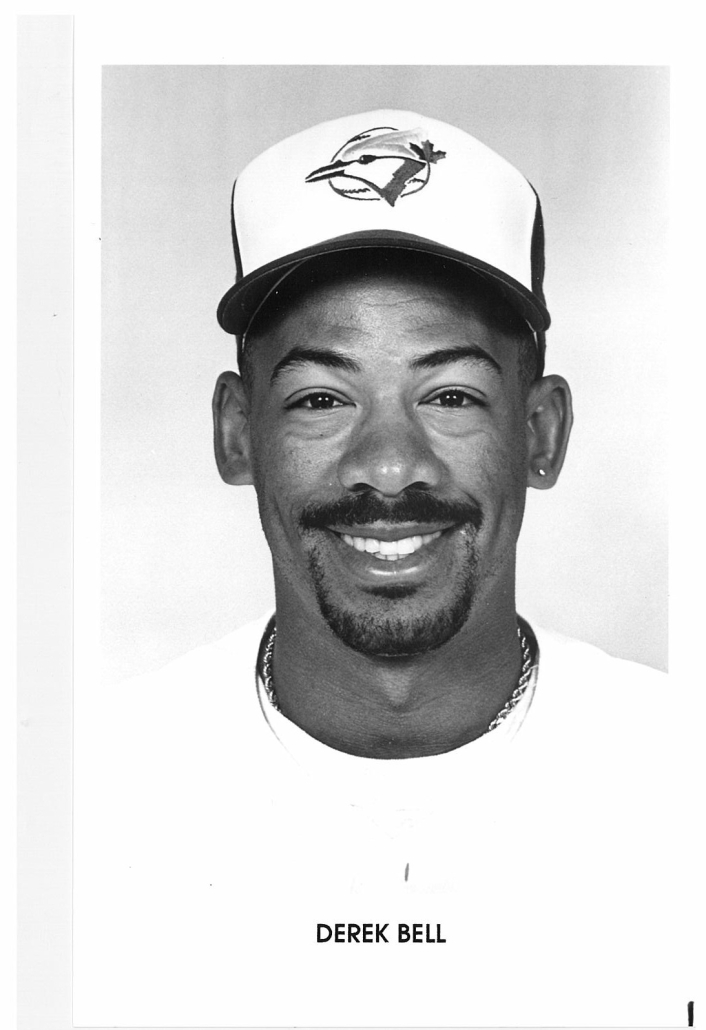This black-and-white head-and-shoulders portrait features Derrick Bell, a baseball player, captured against a subtly illuminated grey background. In the portrait, Bell, an African-American man, smiles warmly, showcasing his mustache and goatee. On his left ear, he wears a light-colored stud earring. He sports a distinctive Toronto Blue Jays cap, characterized by a white front panel and a Blue Jay's head logo looking to the left, contrasted by a darker brim. Bell is dressed in a white shirt that partially conceals a gold necklace around his neck. At the bottom of the image, his name, Derrick Bell, is clearly spelled out in black text.